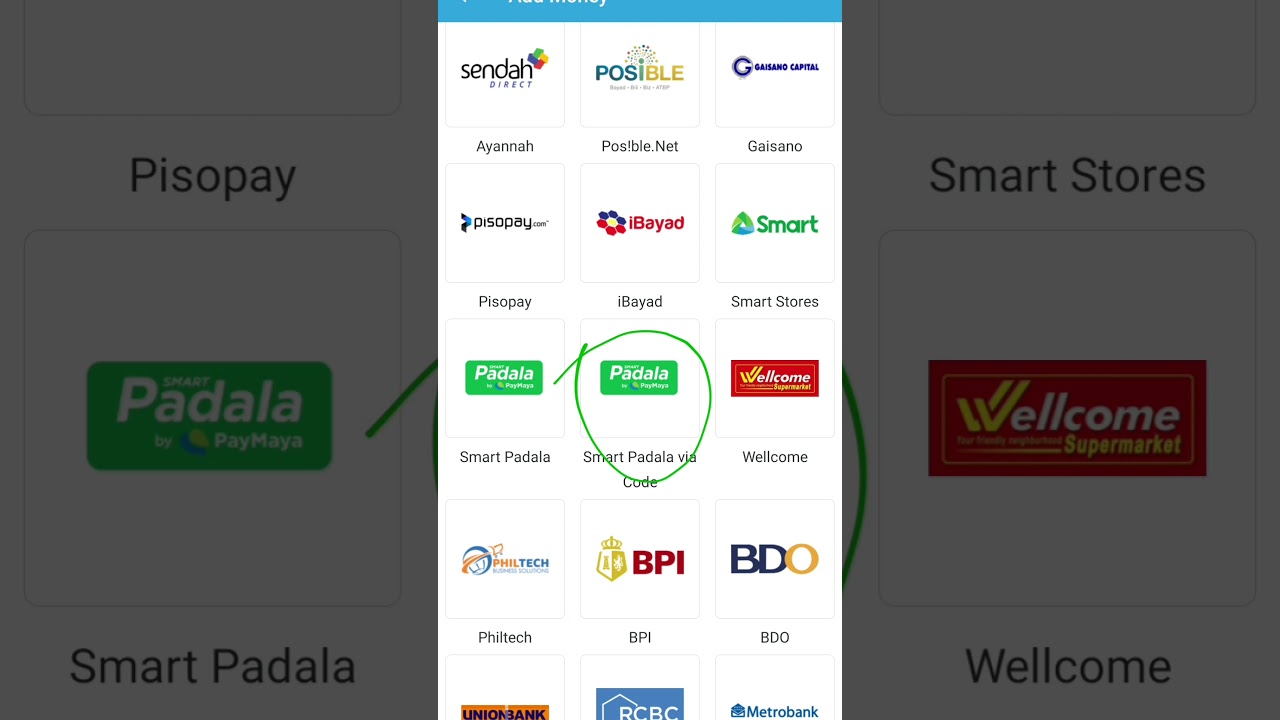In this image, we see a central pop-up menu displaying a variety of buttons to choose from. The buttons are organized into rows with identifiable labels. Starting from the top left, the buttons are labeled as follows: Ayana, thenextispossible.net, Gaisano, PisoPay, iBuyIt, SmartStores, SmartPedala, SmartPedala via code (which is highlighted with a green circle), Welcome, PhilTech, BPI, and BDO. The final row is partially cut off, but the visible icons represent Union Bank, RCBC, and Metro Bank. The background on either side mirrors a zoomed-in section of the central menu: on the left, we see the "SmartPedala" button, and on the right, we see the "Welcome" button, each accompanied by their corresponding symbols from the main menu.